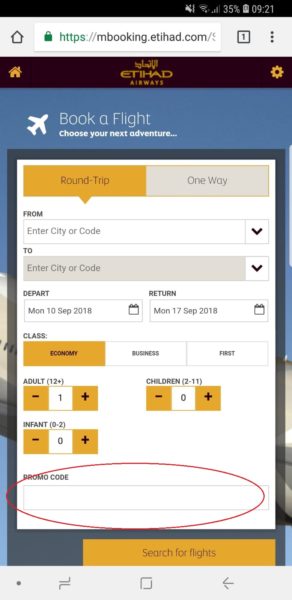Screenshot of a phone showing the Etihad Airways booking page. The phone screen displays the web address "mybooking.etihad.com" in the address bar, which features a home button to the left, a tab button and a context menu to the right. The phone has no sound on, shows four or five bars of signal, Wi-Fi is enabled, and the battery level is at 35% with a time stamp of 9:21.

The main website content is prominently marked with the Etihad Airways logo and the tagline "Book a flight, choose your next adventure," accompanied by a small airplane icon to the left. A bright orange bar indicates 'Round Trip' is selected, with 'One Way' appearing grayed out beside it.

Details of the booking include:
- Departure: Monday, 10th September 2018
- Return: Monday, 17th September 2018
- Class: Economy (with Business and First Class options available but not selected)
- Travelers: 1 adult, 0 children, 0 infants

At the bottom of the booking form is an entry field for a promo code, circled in red. The 'Search for Flights' button is prominent in yellow with black text.

Additionally, the standard navigation buttons - home, back, and menu - are visible at the bottom of the phone screen. Thus, the user is in the process of booking a flight through Etihad Airways.